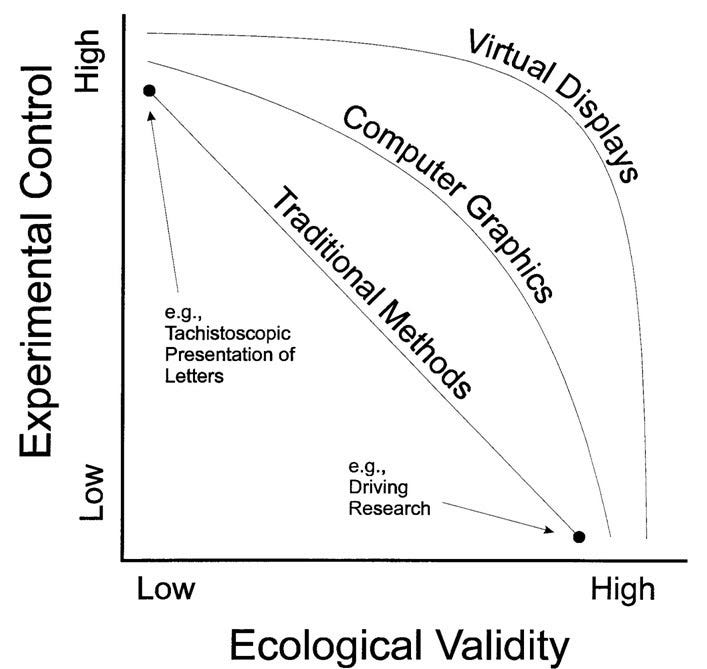This graph illustrates the relationship between ecological validity (x-axis, ranging from low to high) and experimental control (y-axis, also ranging from low to high). The black line, labeled "Traditional Methods," moves steadily from high experimental control and low ecological validity on the left to low experimental control and high ecological validity on the right. Above this, a gently declining line labeled "Computer Graphics" indicates a similar trend but shows a more pronounced drop in experimental control as ecological validity increases. At the very top, another curved line labeled "Virtual Displays" depicts the steepest decline, starting high in control on the left and dropping sharply as it moves right. Arrows point to notable points on the graph; one below "Traditional Methods" reads "Tachoscopic Presentation of Letters," while another on the bottom right end of the line is labeled "Driving Research." The graph is rendered in black and white with clear labels for each axis and plotted line, providing a comprehensive analysis of these different methodologies in terms of their experimental control and ecological validity.